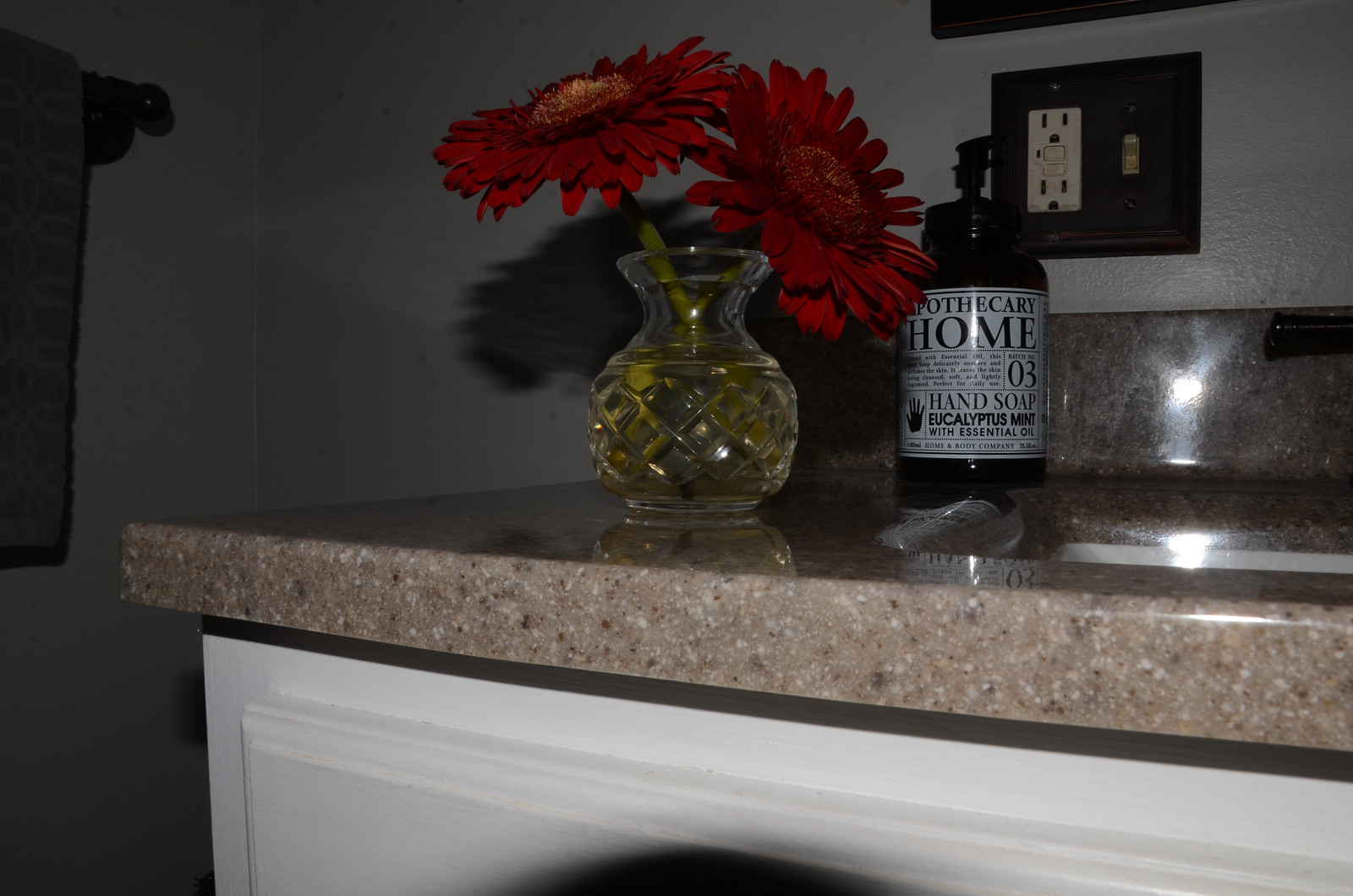A tasteful photograph captures a polished granite countertop with a blend of gray, white, and darker gray flecks, offering a visually appealing texture. Centered on the counter stands a sophisticated clear glass vase with an intricate cut-diamond design, cradling two large, vibrant red flowers with elongated stems that cast elegant shadows against a gray wall backdrop. To the right of this striking floral arrangement sits a sleek, dark-colored jar with a pump top. The jar bears a white label inscribed in black with the name "Apothecary Home" and mentions its contents as hand soap with eucalyptus mint and essential oils, presented by Home and Body Company; the label also features a black-filled drawing of a hand. The countertop, harmoniously extending into a matching granite backsplash, subtly complements the scene. Mounted above the jar with the pump is an electrical outlet paired with a light switch, bordered in black, providing functionality while blending with the overall aesthetic. Further right, the countertop elegantly transitions into a clean and practical sink area.